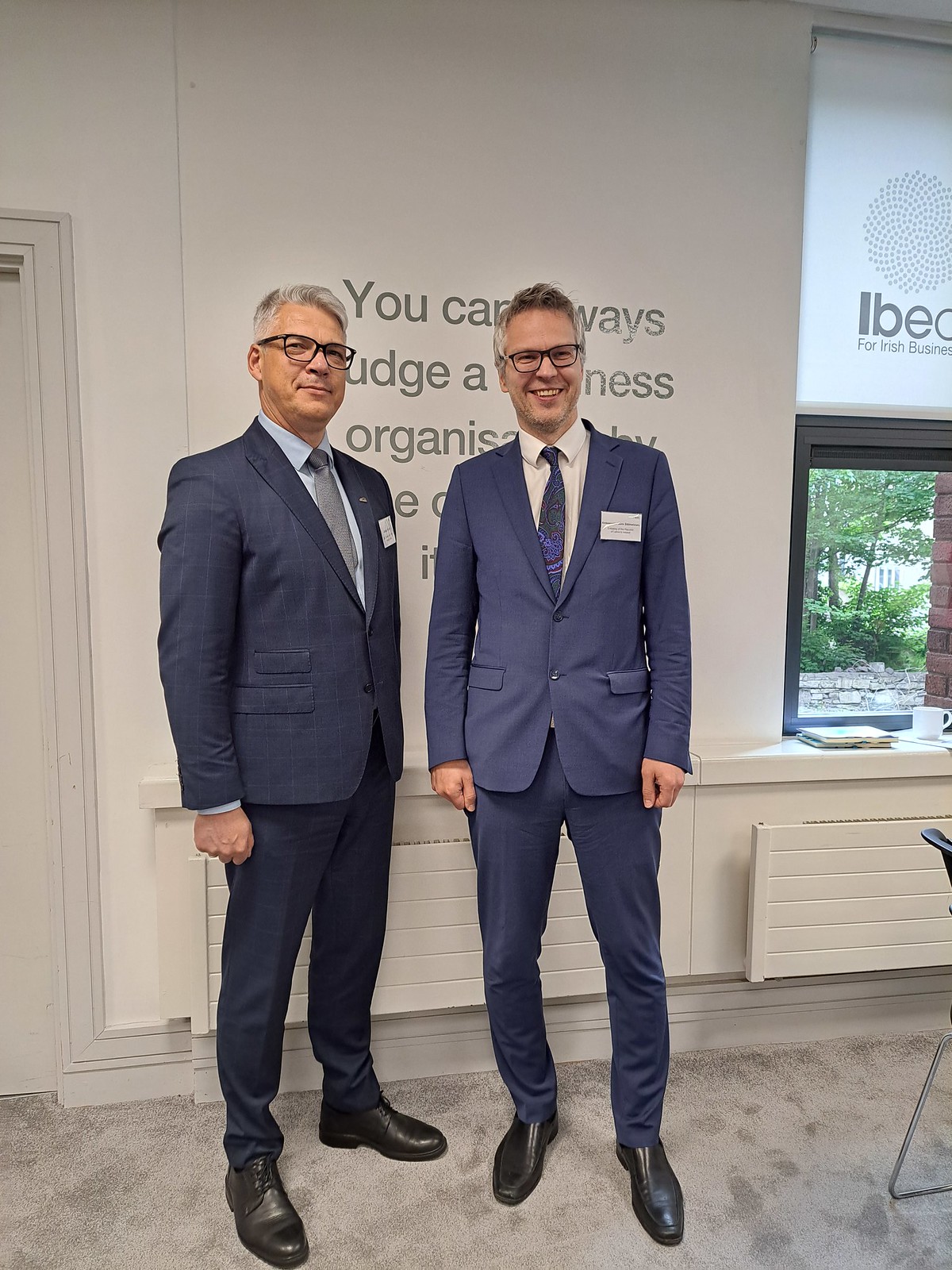The image captures two slender men, likely in their fifties, standing together in what appears to be a meeting room. Both men are dressed in sharp, navy blue suits, complemented by black dress shoes and glasses. The man on the left, exuding a smug look, faces the camera with a grey tie and a name tag barely readable. Meanwhile, the man on the right, adorned with a blue patterned tie, smiles while gazing away from the camera. Both are positioned in front of a white wall featuring an indistinct quote about organization, partially obscured by their presence. The setting includes a window to their left, displaying trees outside, and a partially visible chair within the room. The men stand on a whitish-gray carpet, subtly enhancing the formality of their attire and surroundings.